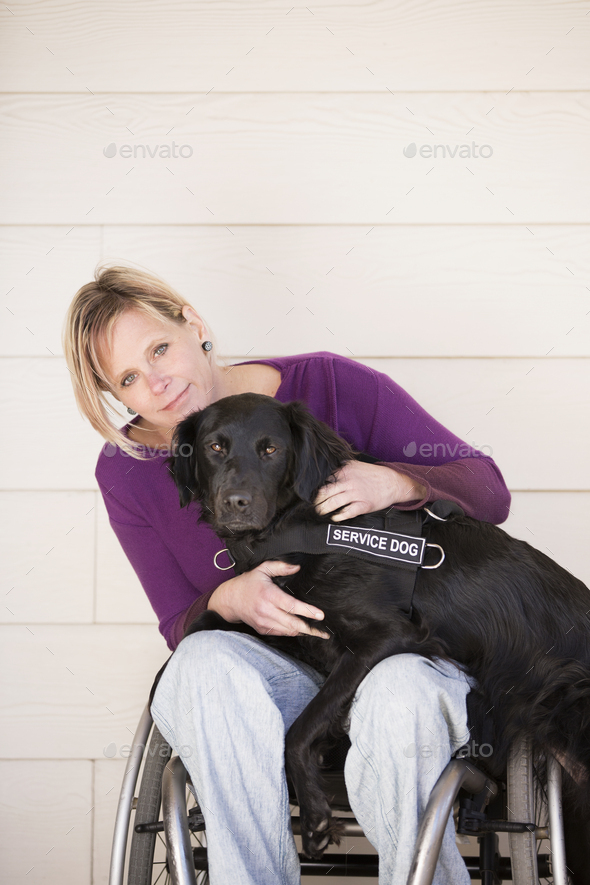The image depicts a young white woman, approximately 30 years old, with dyed blonde hair showing brown roots, dressed in a purple long-sleeve shirt and light blue jeans. She sits in a traditional silver and black wheelchair, leaning slightly forward and to her right. On her lap, a black Labrador retriever, likely a service dog wearing a harness, sprawls with some of its legs on the ground and its body draped across her. The woman hugs the dog, resting her chin lovingly on its head, displaying a content expression. The dog, with a more serious demeanor, gazes directly at the camera. The background features white paneling, and the image bears the watermarked name "Envato" multiple times, indicating it is a stock photograph.